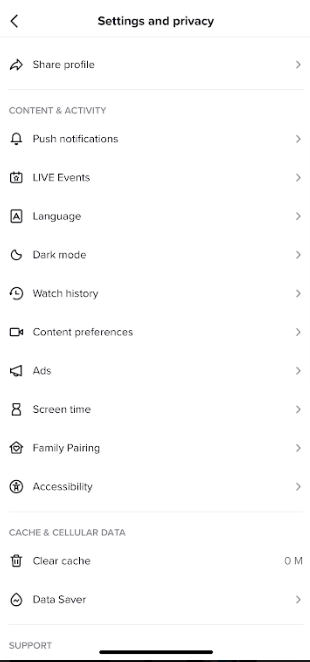Screenshot of a settings page featuring various options in a neatly organized list. The header "Settings and Privacy" is prominently displayed in bold black font, while all other text is in gray. Categories include "Share Profile," "Content and Activity," "Push Notifications," "Live Events" with "LIVE" in all capital letters, "Language," "Dark Mode," "Watch History," "Content Preferences," "Ads," "Screen Time," "Family Pairing," "Accessibility," "Cache," and "Cellular Data." Next to "Clear Cache," a different option featuring a zero, there is an arrow pointing to the right. Below this, "Data Saver" and "Support" appear. A black rectangle is located in the bottom middle of the screen.